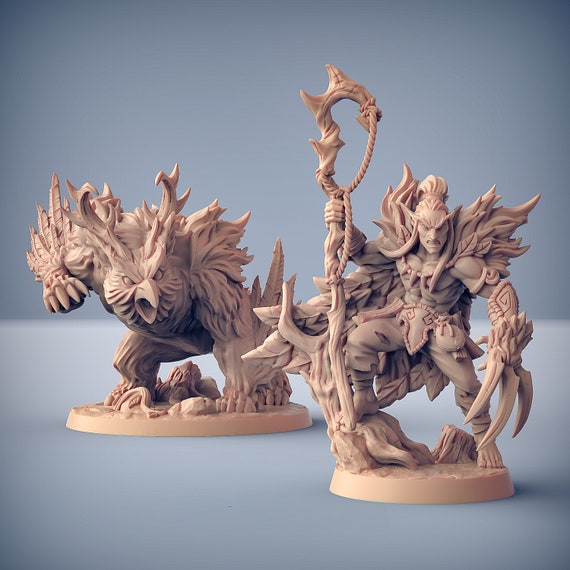This image showcases two intricately designed figurines against a light gray background adorned with shadowing. Both figurines are made of a tan, light brown material, giving them a cohesive look. On the left, there is an animal-like creature with a pronounced beak wide open in a snarling expression, adorned with stag-like horns and feathers. It has five finger claws on its right hand, which seems to be in motion, while its left hand rests on the surface, possibly touching something on the ground.

On the right side, the figurine depicts a man heavily armored, standing in a dynamic pose with one foot elevated on a rock. This figure is equipped with a large claw-like glove on one arm and wields a sizable staff or hook with a rope in the other. The man has long hair flowing down, adding to his imposing presence, and he features wings, enhancing the fantastical element of the sculpture. Together, these figurines create a striking, detailed scene of mythological intrigue.